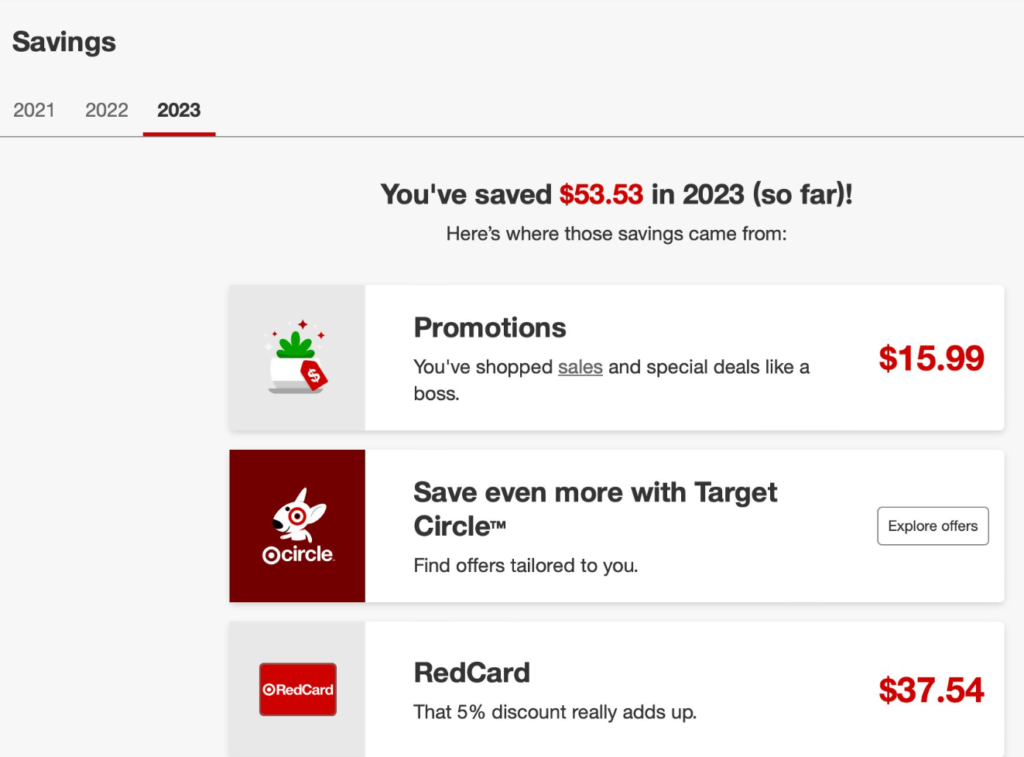This is a detailed description of a webpage dedicated to savings on a personal website. 

At the top of the page, there is a heading that reads "Savings." Below this, there are navigational tabs labeled for different years: 2021, 2022, and 2023, with the current year, 2023, being highlighted. Directly underneath the tabs, a thin light gray line is followed by the text: "You've saved $53.53 in 2023 (so far!)". This indicates the total savings accumulated in the current year.

Further down the page, there is a visual representation of the savings. The image depicts a green plant in a flower pot with three stars hovering above it and a dollar sign tag hanging from it, suggesting financial growth or savings. 

To the right of this image, in a slightly grayish-white box, is a section titled "Promotions." The text reads: "You've shopped sales and special deals like a boss," followed by the savings amount of "$15.99" underlined to emphasize the sales. 

Below the promotions section is another segment showcasing a circular icon with an illustration of a pit bull with a circle around its left eye, set against a burgundy background. To the right of this icon, in another white box, are the words: "Save even more with Target Circle. Find offers tailored to you," with a prompt button labeled "Explore Offers."

Lastly, the page includes information about savings with a red card. This section features an image of a red card with white text that reads "REDcard." To the right, in a white box, it states: "That 5% discount really adds up," amounting to a total saving of "$37.54."